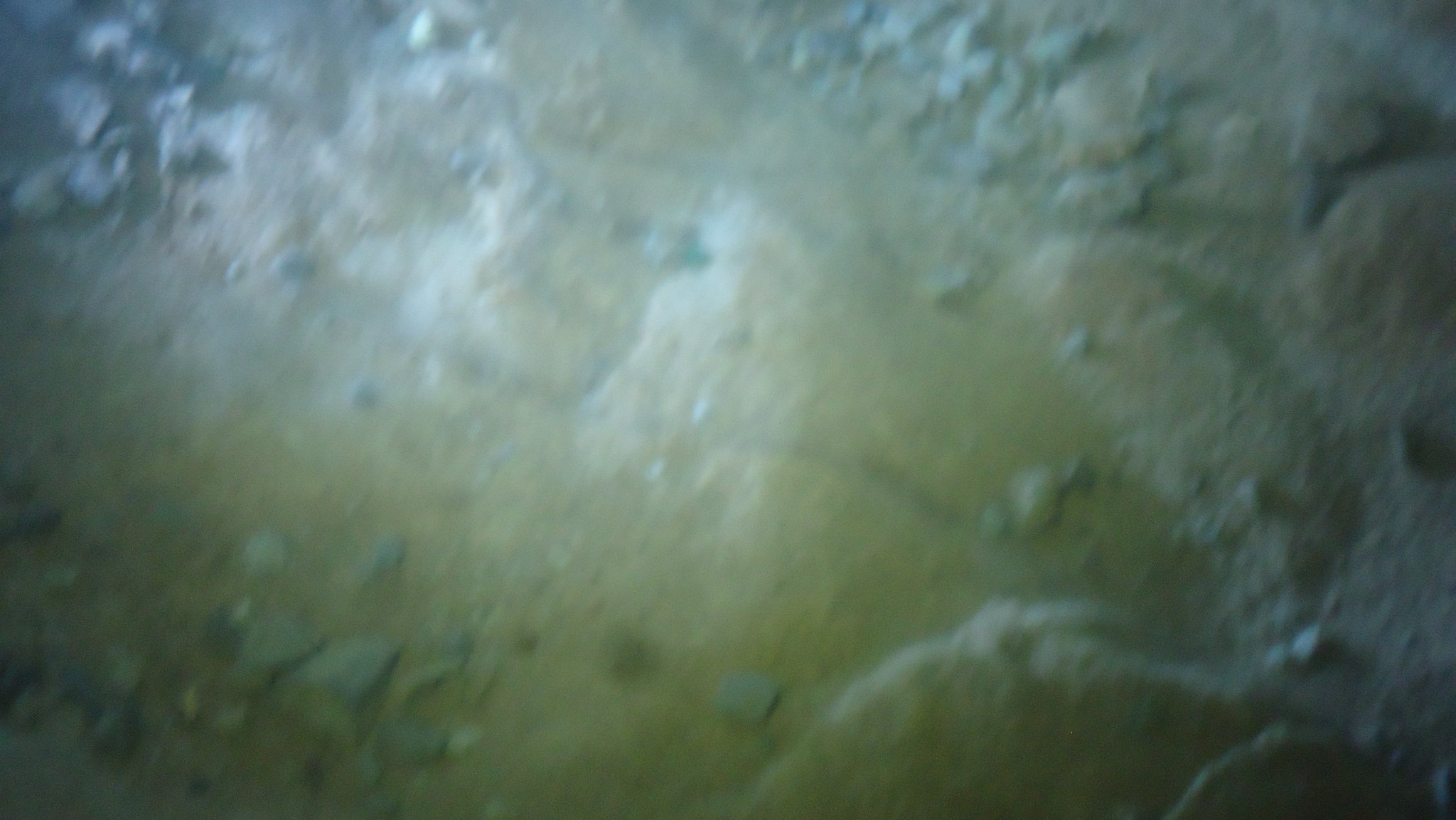This nighttime photograph, possibly taken outdoors with a flash camera, showcases the ground illuminated in the upper left-hand corner. The surface appears uneven, with small mounds of dirt complemented by scattered sharp-edged, gray rocks. These rocks are concentrated primarily in the lower left-hand corner, upper left-hand corner, and center-right of the image. The remaining area features a more uniform, flat expanse of dirt with occasional rounded patches. The contrasting textures between the dirt and rocks create a rugged landscape, starkly highlighted by the camera's flash in the dark night.